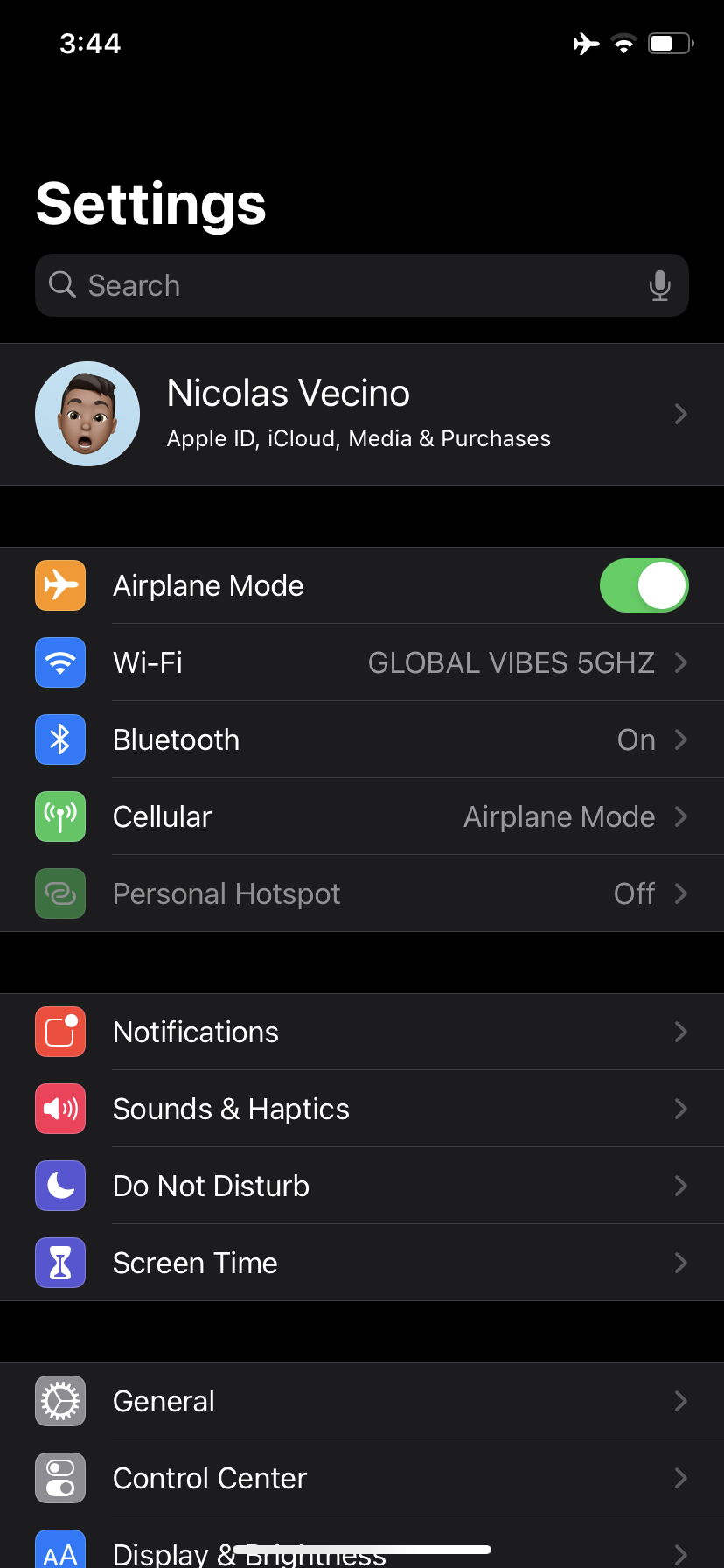Screenshot of a Phone's Settings Page on Airplane Mode

This detailed screenshot captures a phone's settings page with a sleek black background. At the very top of the screen, the number "344" is displayed, suggesting either the time or a specific notification count. Alongside it, there are icons for airplane mode, Wi-Fi, and battery status.

The header, “Settings,” is prominently displayed in bold white font, just below which is a search bar for easy navigation. Below the search bar, there's a profile section featuring a cartoon avatar of a man with his mouth open, labeled "Nicholas Vecino," followed by links to Apple ID, iCloud, media, and purchases.

The settings options are listed as follows:

1. **Airplane Mode** - Toggled to "On."
2. **Wi-Fi** - Connected to "Global Vibes 5GHZ."
3. **Bluetooth** - Turned on.
4. **Cellular** - Disabled due to airplane mode.
5. **Personal Hotspot** - Set to "Off."
6. **Notifications**
7. **Sounds & Haptics**
8. **Do Not Disturb**
9. **Screen Time**
10. **General**
11. **Control Center**
12. **Display & Brightness**

Each option is accompanied by a uniquely colored icon, including shades of orange, blue, green, red, purple, and gray, providing a visually appealing layout.

At the bottom of the screen is a long white bar, which is likely the home indicator for gesture navigation. This clean and detailed layout offers a comprehensive view of the phone's current settings and status.